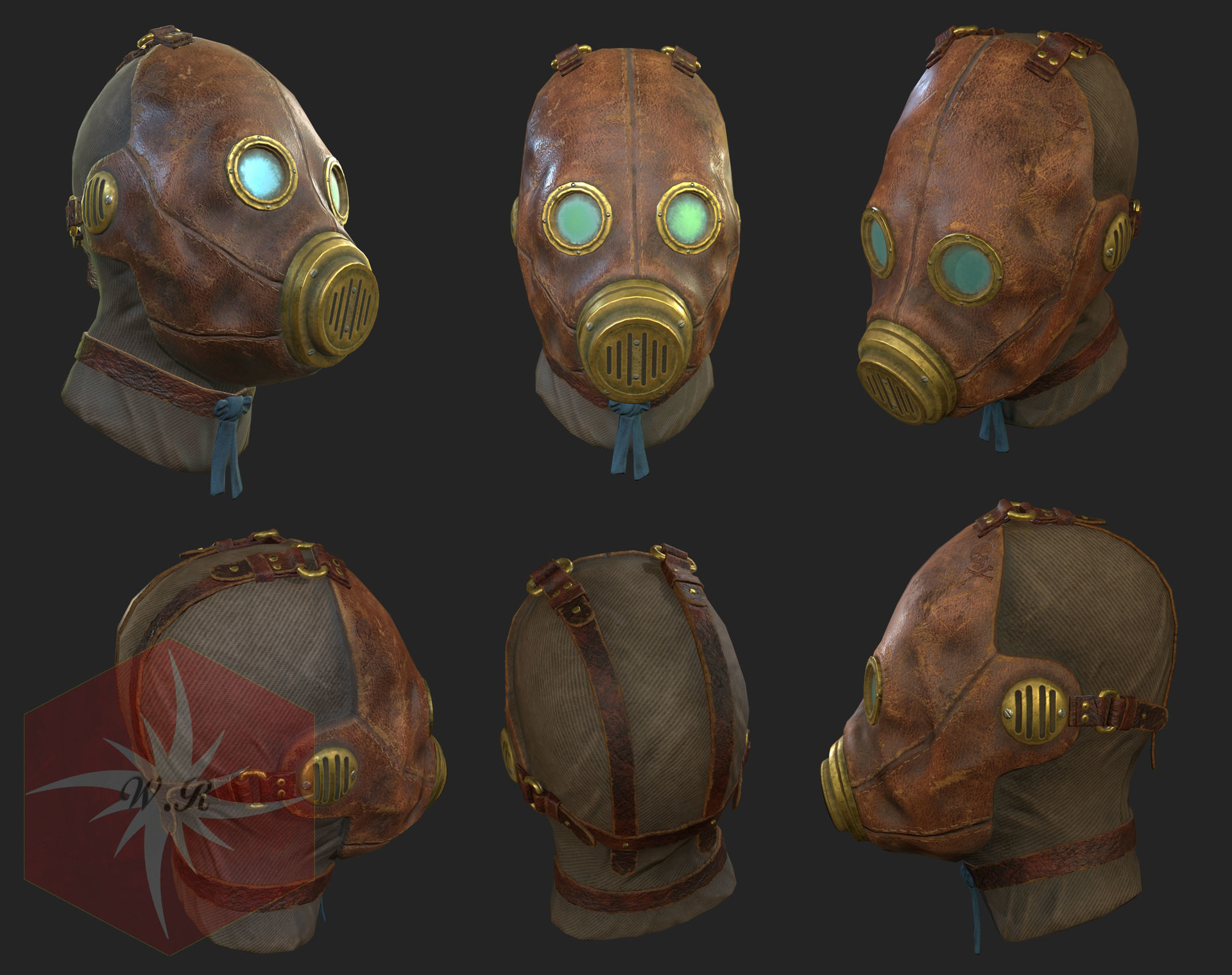This illustration showcases six different angles of a CGI character's head wearing a detailed, old-style gas mask. The mask is predominantly made of brown leather and is adorned with brass features, including ringed eyelets around green-tinted glass goggles, a brass respirator over the mouth, and vented brass slits over circular ear coverings. The head of the CGI character is fully covered in a cloth or mesh material, obscuring any details of what lies beneath. Straps made of brown leather, fastened by brass buckles, secure the mask with two straps going over the top of the head and one around the back. The character also wears a matching brown leather collar with a blue ribbon. The image is arranged to display front, back, left and right side perspectives, drawing attention to the meticulous design and functional aspects of the gas mask. Additionally, a distinctive detail in the bottom left corner includes the letters "W.R." inside a red star-like symbol.